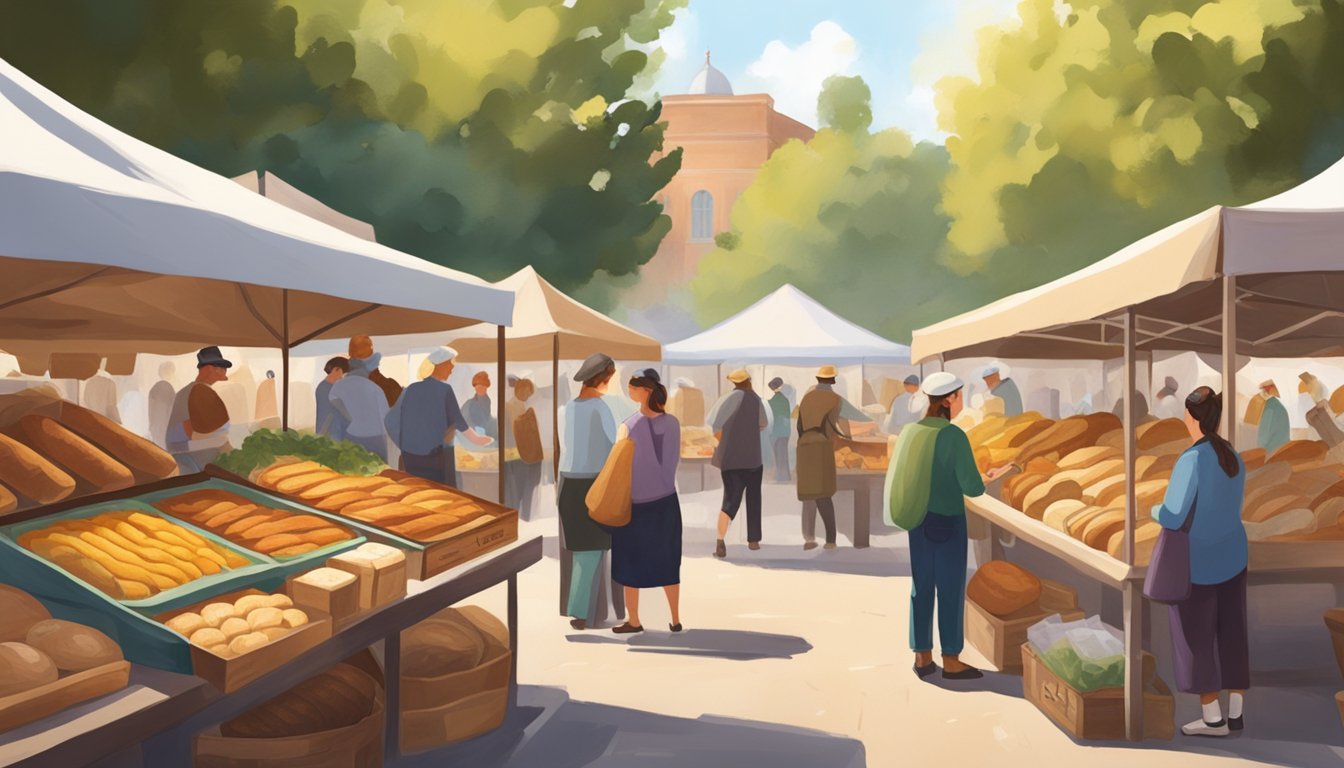This illustration, created in a computer-generated, cartoon-style with an impressionist touch, depicts a bustling street market scene reminiscent of a downtown farmer's market. The market is set up along a stone-paved walkway, flanked by rows of white and tan tents that house various vendors and their goods. The foreground tents, brimming with an impressive variety of bread loaves, display rolls and long, artisan-style breads. On the opposite side, additional tents are laden with baked goods, where two ladies are examining large pieces of cheese or bread.

The market is alive with numerous people strolling through the walkways, many of them carrying bags and dressed in colorful attire. Among the shoppers, notable figures include men in blue shirts and different colored hats, and a lady wearing a purple top with a blue skirt. The shoppers seem engrossed in the offerings, which speaks to the market’s vibrant atmosphere. Overhead, green trees provide a natural canopy, adding to the inviting ambiance. In the background, a partially visible brick building with a single window hints at the quaint charm of the surrounding architecture. The overall impression of this scene is one of community and lively commerce, captured through blurred, yet vivid, artistic details.